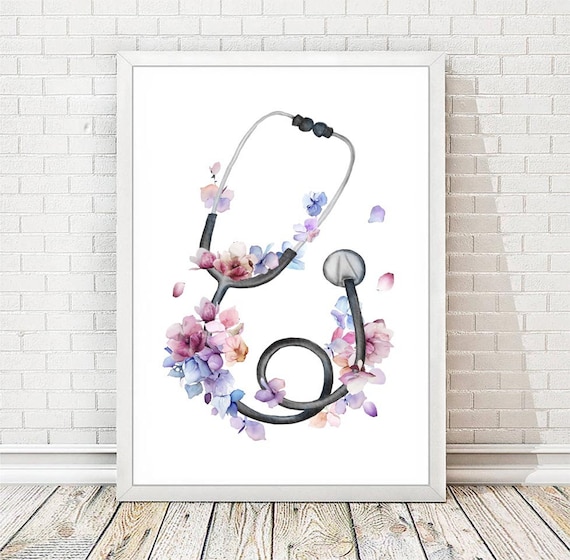This vertical rectangular digital artwork, set against a backdrop of white brick walls and a light, grayish wooden floor, features a large white framed painting leaned against the wall. A white baseboard runs along the bottom of the wall, adding to the setting's clean aesthetic. The focal point of the painting is a stethoscope, depicted at an angle with the earpieces oriented around a one o'clock position, if visualized as a clock. The stethoscope itself has black rubber pieces on the ends and a mixture of gray and black parts along its length. It loops gracefully at the bottom, and the chest piece rests near the upper section. The most striking element of the image is the array of flower petals adorning the stethoscope. These petals, in shades of blue, purple, red, pink, light brown, and a hint of orange, are scattered generously across the medical device, providing a vivid contrast to the white background. This harmonious blend of medical precision and natural beauty creates a very captivating and serene composition.